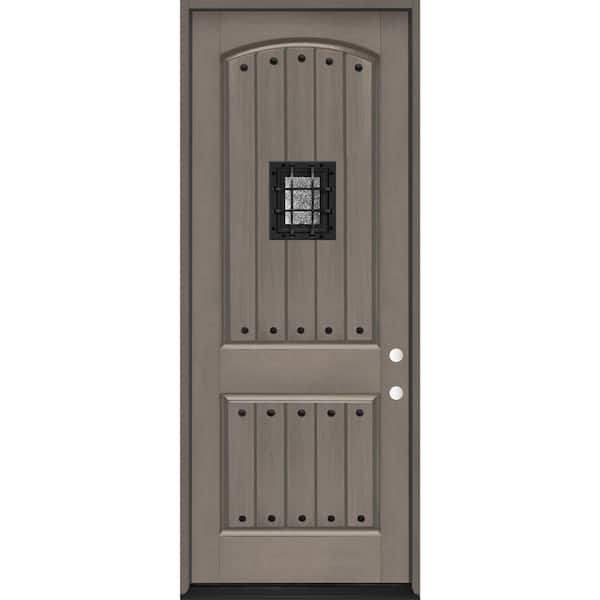The image features a digitally-created, rectangular gray door positioned centrally against a completely white background. This door, which takes up about two-thirds of the image, is enclosed within a slightly darker gray frame. The door itself is divided into two sections: the top section occupies two-thirds of the door and houses a rectangular glass window crisscrossed with black metal bars resembling a tic-tac-toe pattern. Both sections of the door have five vertical panels, with each panel topped and bottomed by black circular knobs. Additionally, the right side of the door features two white circles, about one-third up from the bottom, representing the doorknobs. The overall composition gives the impression of an illustrated representation rather than a real door.